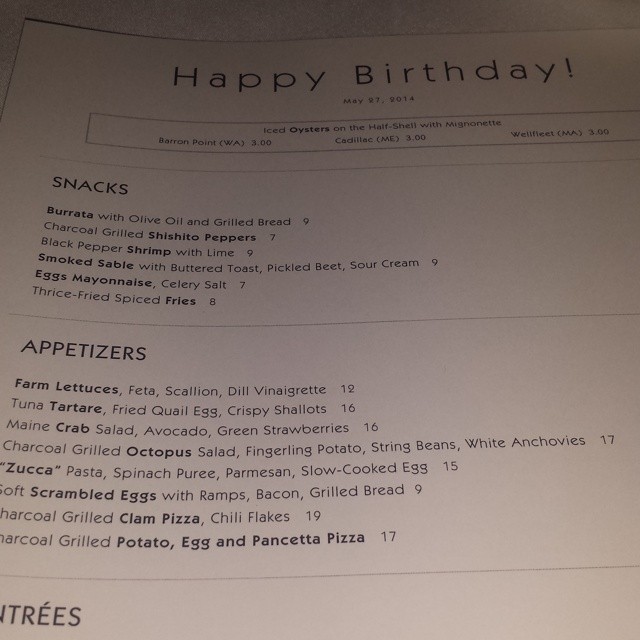A detailed menu displayed on a white piece of paper, resting on a white table, is headed with "Happy Birthday!" in large black letters, dated May 27th, 2014. Below the heading, a light gray-outlined vertical box lists "Iced oysters on the half shell with mignonette," specifying varieties such as Baron Point, Cadillac, and Wellfleet. Following this, "Snacks" is prominently featured with entries like "Burrata with olive oil and grilled bread ($9)," "Charcoal grilled shishito peppers ($7)," "Black pepper shrimp with lime ($9)," "Smoked sable with butter toast, pickled beet, sour cream ($9)," "Eggs mayonnaise or celery salt ($7)," and "Thrice fried spiced fries ($8)," with the main ingredients bolded. A light gray line separates the snacks from the "Appetizers," which include items like "Farm lettuce with feta, scallion, dill vinaigrette ($12)," "Tuna tartare with fried quail egg and crispy shallots ($16)," "Maine crab salad with avocado and green strawberries ($16)," "Charcoal grilled octopus salad with fingerling potato, string beans, white anchovy ($7)," "Zucca pasta with spinach puree, Parmesan, slow-cooked eggs ($15)," "Soft scrambled eggs with ramps, bacon, grilled bread ($9)," "Charcoal grilled clam pizza with chili flakes ($19)," and "Charcoal grilled potato, egg, and pancetta pizza ($17)." The section for "Entrees" is mentioned at the bottom, but is partially cut off.